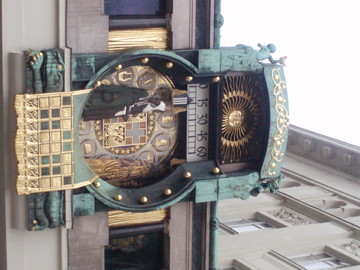In the background of the image, there's a cream-colored stone building, potentially captured from an unusual angle — either sideways or upside-down. The structure is visually appealing with visible architectural details, including two windows. Adjacent to the building, there's an intricate, green clock adorned with gold accents. The clock face displays markings at 15, 30, 45, and 60, with a stationary dial pointing to 15. The combination of the building's classic aesthetic and the ornate clock creates a unique and charming scene.